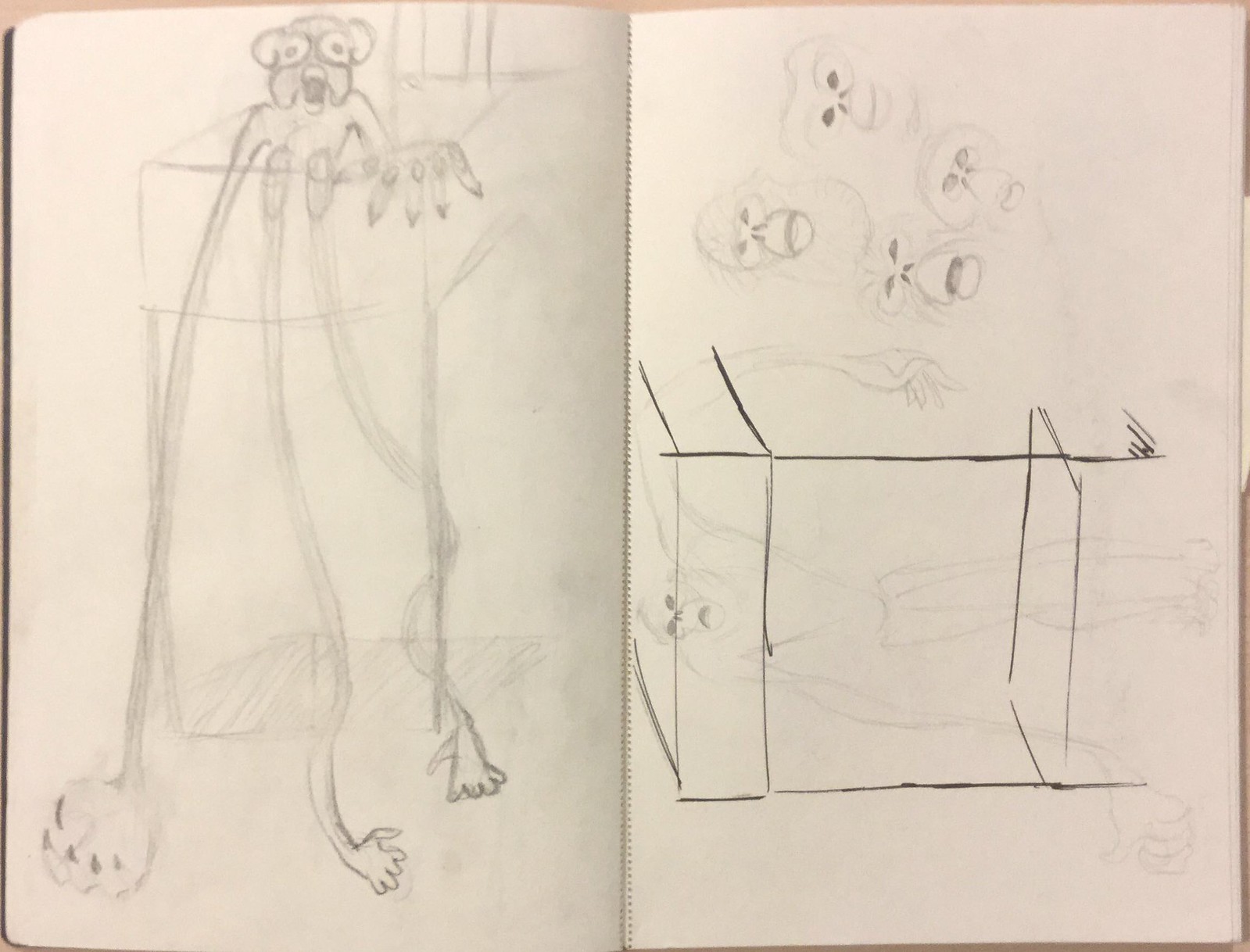The image presents an open drawing pad showing two distinct child's drawings on separate pages, separated by a vertical crease running from top to bottom. On the left page, a bizarre, deranged monkey with exaggerated features is depicted. This monkey has incredibly long, spaghetti-like limbs, with one elongated hand curving upwards, revealing its palm and long claws. The other hand, positioned around a tub or platform from which the monkey appears to emerge, showcases visibly pronounced knuckles. Its face is chaotic, with a gaping mouth and large, crazy eyes that almost resemble spectacles due to their bordered outline. The feet are simplistic and cartoonish, adding to the strange, unsettling vibe of the drawing.

The right page contrasts with a more detailed and realistic illustration of monkey faces and other elements. In the foreground, a faintly erased figure of a muscular monkey man is barely visible, with only his face prominently remaining. Above this figure, there are four disembodied monkey heads, each displaying a unique facial expression: happiness, distress, a human-like face with a large nose, and a skull-like frown. These heads appear to be concept sketches, adding an eerie disjointedness to the overall composition. The page also includes a lightly sketched tray structure, contributing to the mysterious atmosphere of the drawings.